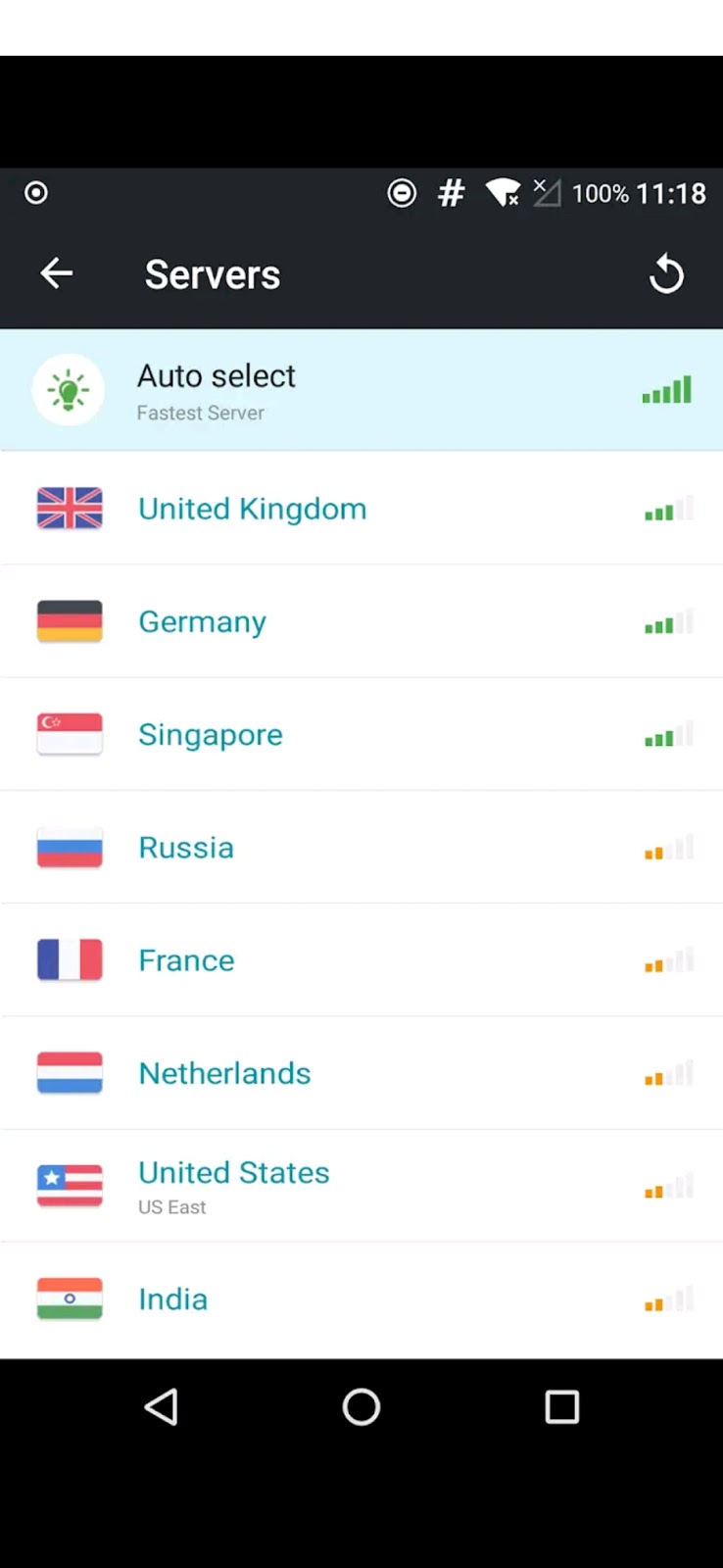At the top of the image, there is a black bar featuring several icons: a large circle symbol, a pound sign, a Wi-Fi symbol indicating no signal, and a 100% battery life indicator. The time displayed is 11:18. To the left, there's an arrow pointing left, labeled "servers," and a pair of circular arrows, likely representing refresh or sync options. In the center, there's a white circle, reminiscent of a green lightbulb icon, and an "auto-select" option is indicated beside it.

Below this, a series of flags and signal strength bars are displayed:

- The United Kingdom flag, in red and blue, accompanied by five green bars.
- The Germany flag, in black, red, and yellow, with three green bars.
- The Singapore flag, in white, blue, and red, along with two yellow bars.
- The France flag, in blue, yellow, and red.
- The United States flag, predominantly blue, with alternating red and white stripes.
- The India flag, featuring red, white, and green.

At the bottom of the image, there's a black section containing a circle and a square symbol.